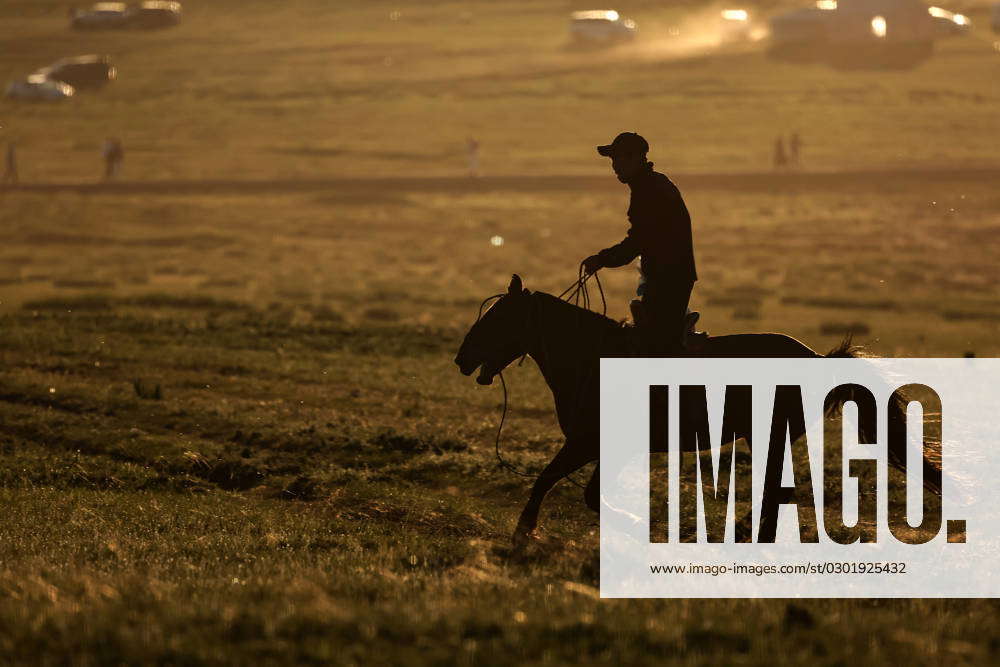This photograph captures the striking silhouette of a man riding a horse in a dimly lit field, either at dawn or dusk, as no colors are visible in the image. The rider is attired in a hat and a long sleeve shirt, appearing to stand rather than sit on the horse, gripping the reins firmly. The horse itself has large ears and an open mouth, suggesting movement and energy. The background reveals a sprawling ranch landscape with numerous buildings, a truck, and possibly other riders, albeit faint and indistinguishable due to the image's small scale. Dust and dirt cloud the area, adding texture to the scene. Large logos marked as "IMAGO" and a URL (www.inigo.images.com/st/0301925432) indicate the source of the photograph. The low lighting, likely from a setting or rising sun, casts a dramatic, almost filmic atmosphere over the entire composition.